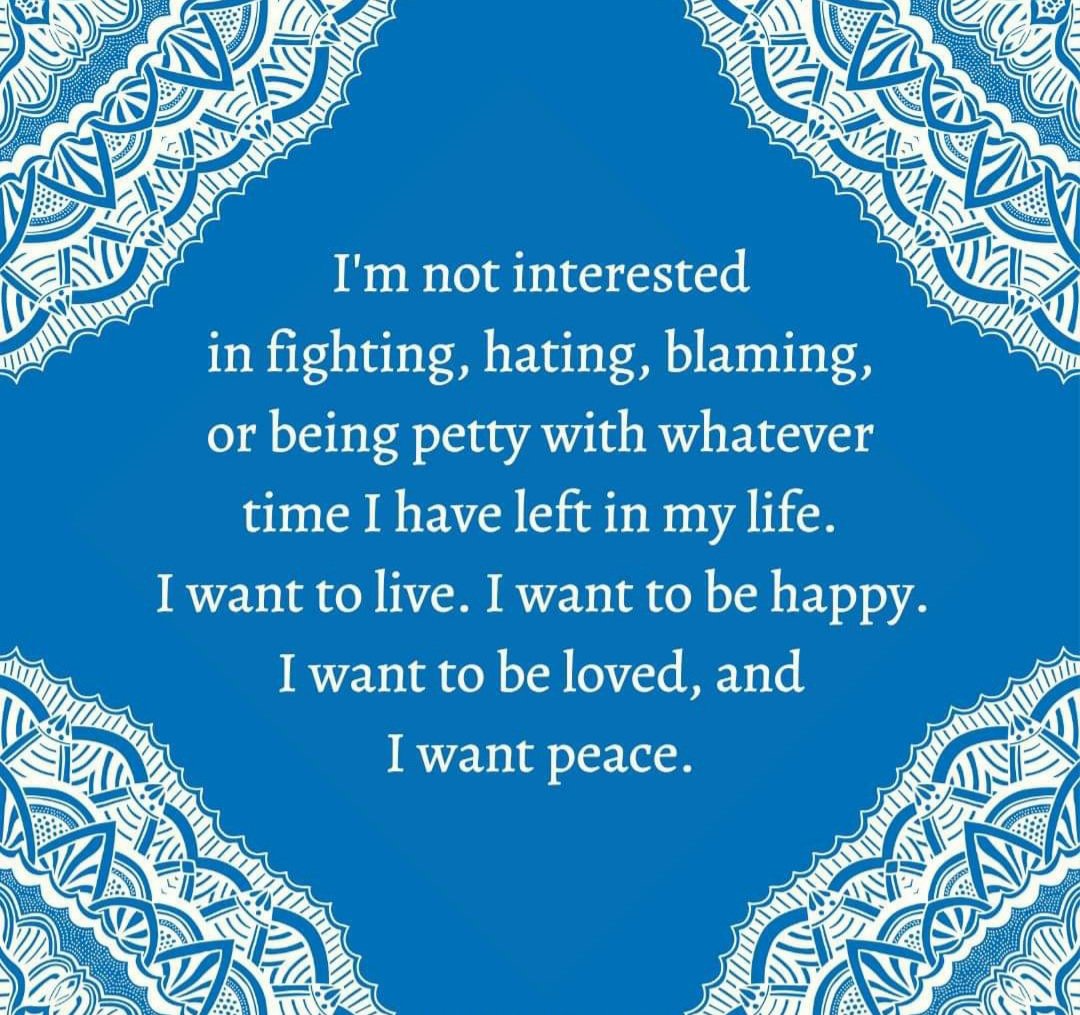The image features a text-based quotation prominently displayed against a blue background. The text itself is in a white font and centered within the image, elegantly formatted across seven lines. The quote reads, "I'm not interested in fighting, hating, blaming, or being petty with whatever time I have left in my life. I want to live, I want to be happy, I want to be loved, and I want peace." Adding to the visual appeal, the corners of the image are adorned with intricate, wavy patterns resembling lace. These decorative elements, which include arches, triangles, waves, stripes, and petal-shaped designs, create a beautiful framework around the central text. The image captures the essence of an "insipid wisdom quote" commonly seen on social media platforms like Facebook, often posted by someone seeking to share positive sentiments.